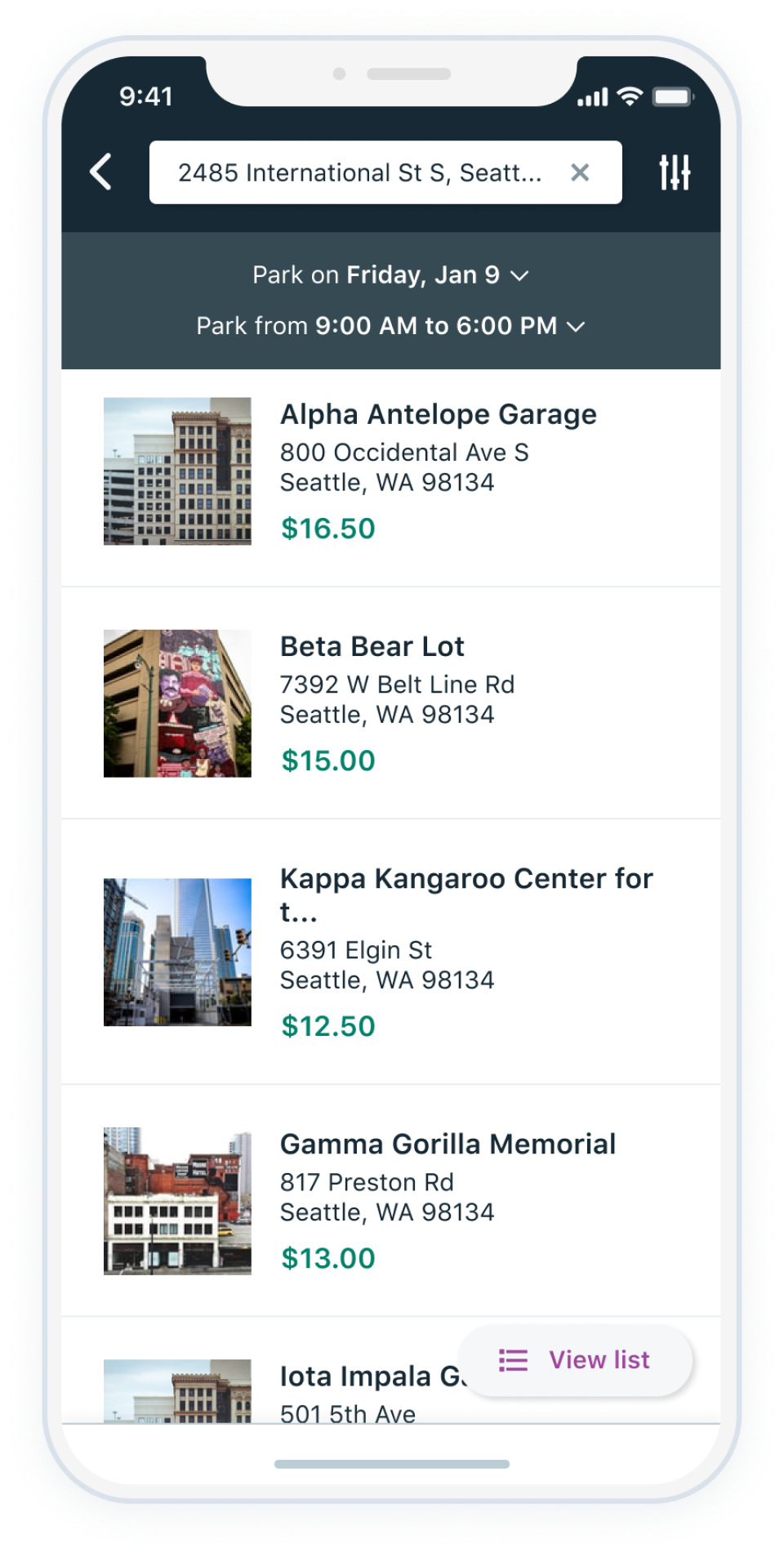This image presents the search results displayed on a cartoon or artificially illustrated cell phone screen. The photograph itself captures a real screen, but the external border of the phone is sketched to simulate its appearance within a drawn device. The phone's frame is white, with a rectangular shape featuring rounded edges and a distinctive black border running horizontally across the top, displaying the time "9:41." Below this, a white search bar with black text reads "2485 International Street S Seattle," though it is partially cut off, followed by filter options on the right.

The phone is oriented in portrait mode, significantly longer than it is wide. Beneath the search bar, the display features a gray border stating "park on January 9th" with a dropdown arrow, and "park from 9am to 6pm" with another dropdown arrow. This section is followed by search results, each separated by thin grayish-black horizontal lines.

The first search result lists "Alpha Antelope Garage" priced at $16.50, accompanied by a thumbnail image of a building. Next is the "Beta Bear Lot" with a price of $15. Following this is an entry that reads "Catholic Kangaroo Center for T," which is cut off, priced at $12.50. The fourth result is "Gamma Gorilla Memorial" listed at $13, with some details cut off mentioning something about "in Piota and Paliton." At the bottom right of the listings is a "view list" button, displayed in purple font within a white oval.